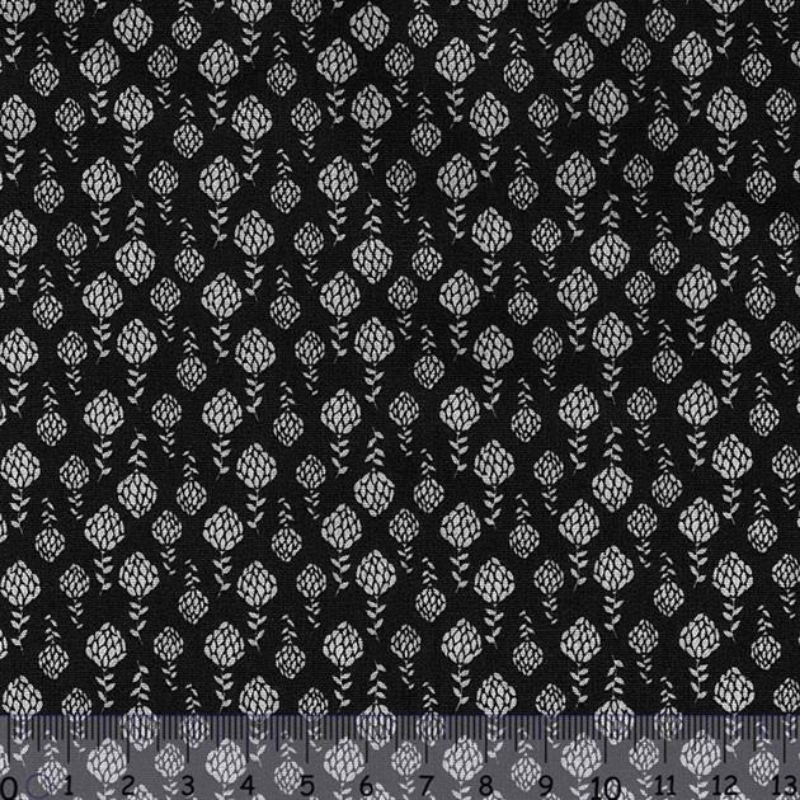This image features a repetitive wallpaper or fabric design set against a stark black background. The pattern consists of white plant motifs that resemble flower buds or small bulbs with stems and leaves. The pattern is meticulously arranged in geometric rows and columns, with larger motifs interspersed with smaller ones, some oriented upside down to create visual variety. The black background contrasts sharply with the white botanical elements, making the pattern stand out. Spanning the bottom of the image is a semi-transparent, opaque ruler marked from 0 to 13, likely representing centimeters, which provides a scale for the dimensions of the pattern. This ruler is white with black text and lines, helping to contextualize the size of the design elements within the image.